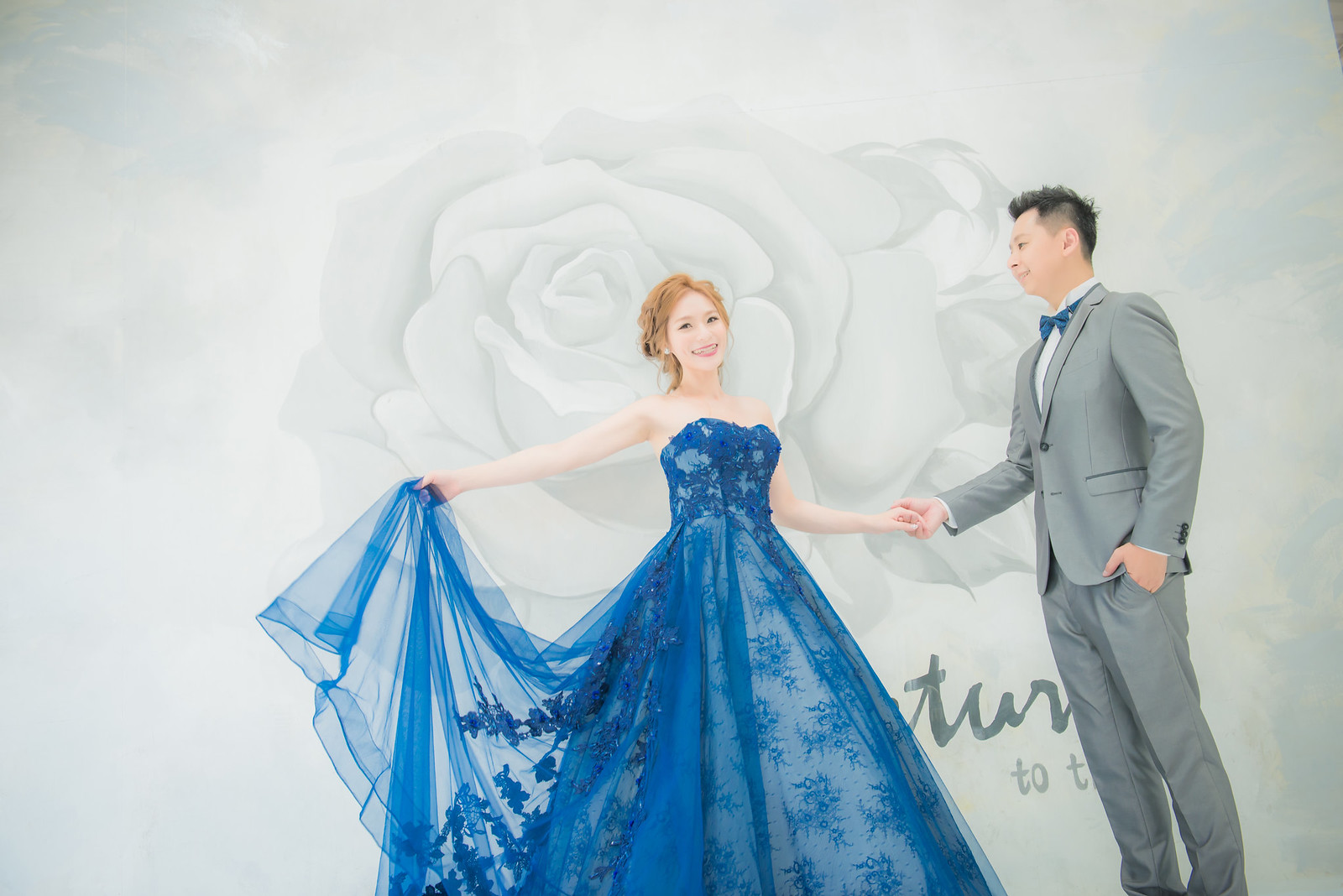In this black and white image, a young Asian couple is seen posing in front of a textured backdrop featuring a painted grey rose and some text that is partially covered by their figures. The woman, who has reddish, almost orange hair, is dressed in a strapless blue gown. Her gown is sheer over a simpler white dress, and she elegantly holds out the train with her right hand. She holds her partner's hand with her left hand while smiling radiantly. The man, standing to her right, is wearing a sharp gray suit complemented by a white shirt and a blue bow tie that perfectly matches her dress. He has short, dark hair and keeps one hand casually in his pocket, smiling warmly at the camera. The couple's joyful expressions and synchronicity in their attire evoke a sense of celebration, suggesting they might be at a formal event such as a prom or perhaps engaged in a themed photo shoot rather than a wedding, given their youthful appearance.